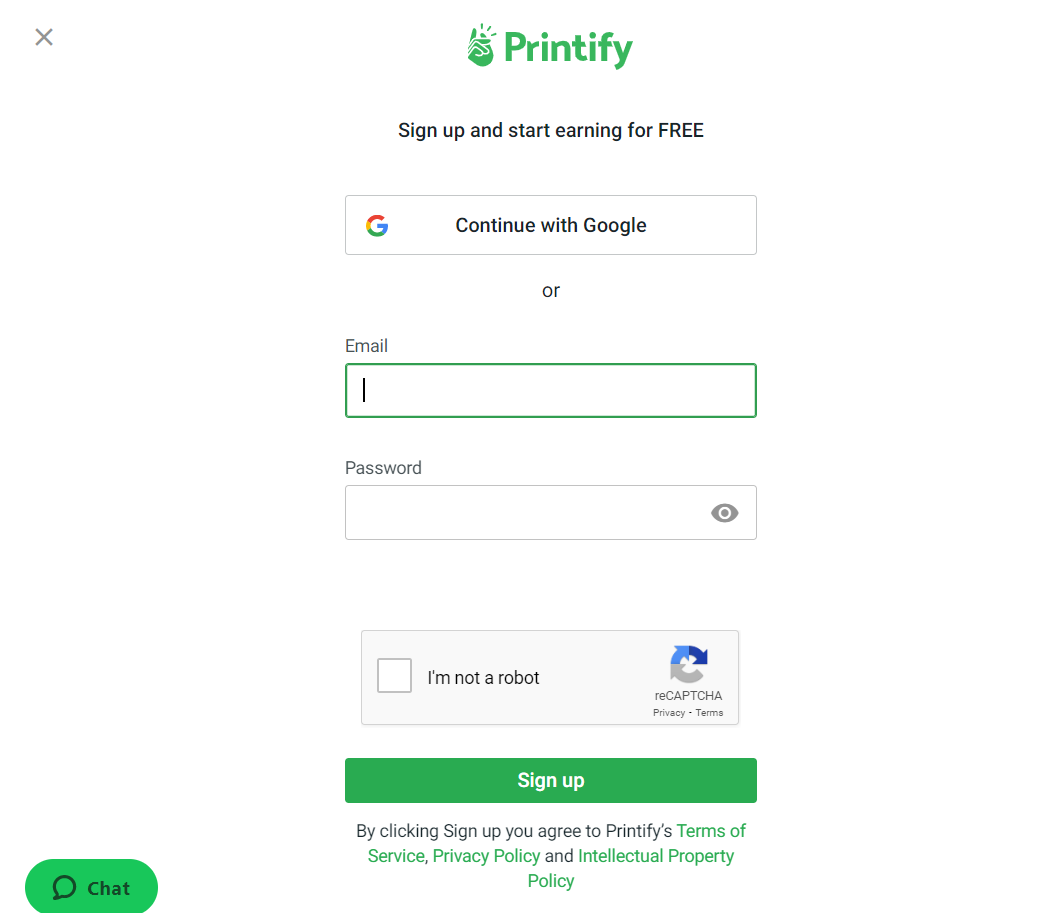This image is a screenshot from the mobile version of the Printify app, displayed on a white background. At the top center, the word "Printify" is written in green letters next to a green hand icon making a snapping gesture with three lines above the fingers to indicate sound or motion. Below this, the text reads, "Sign up and start earning for free."

Underneath the introductory text, there's a box featuring the Google symbol on the left, which invites users to "Continue with Google" for a simplified sign-up process. Below this box, the word "or" appears in black, directing users to alternative sign-up options. The image then shows fields for entering an email address and a password of the user's choice.

Further down, there's a reCAPTCHA verification where users tick a box next to the statement "I'm not a robot." Positioned below this verification is a green "Sign Up" button. In the lower-left corner of the screen, a green chat button is available for users to initiate a conversation with customer service. The sign-up terms are displayed beneath the "Sign Up" button.